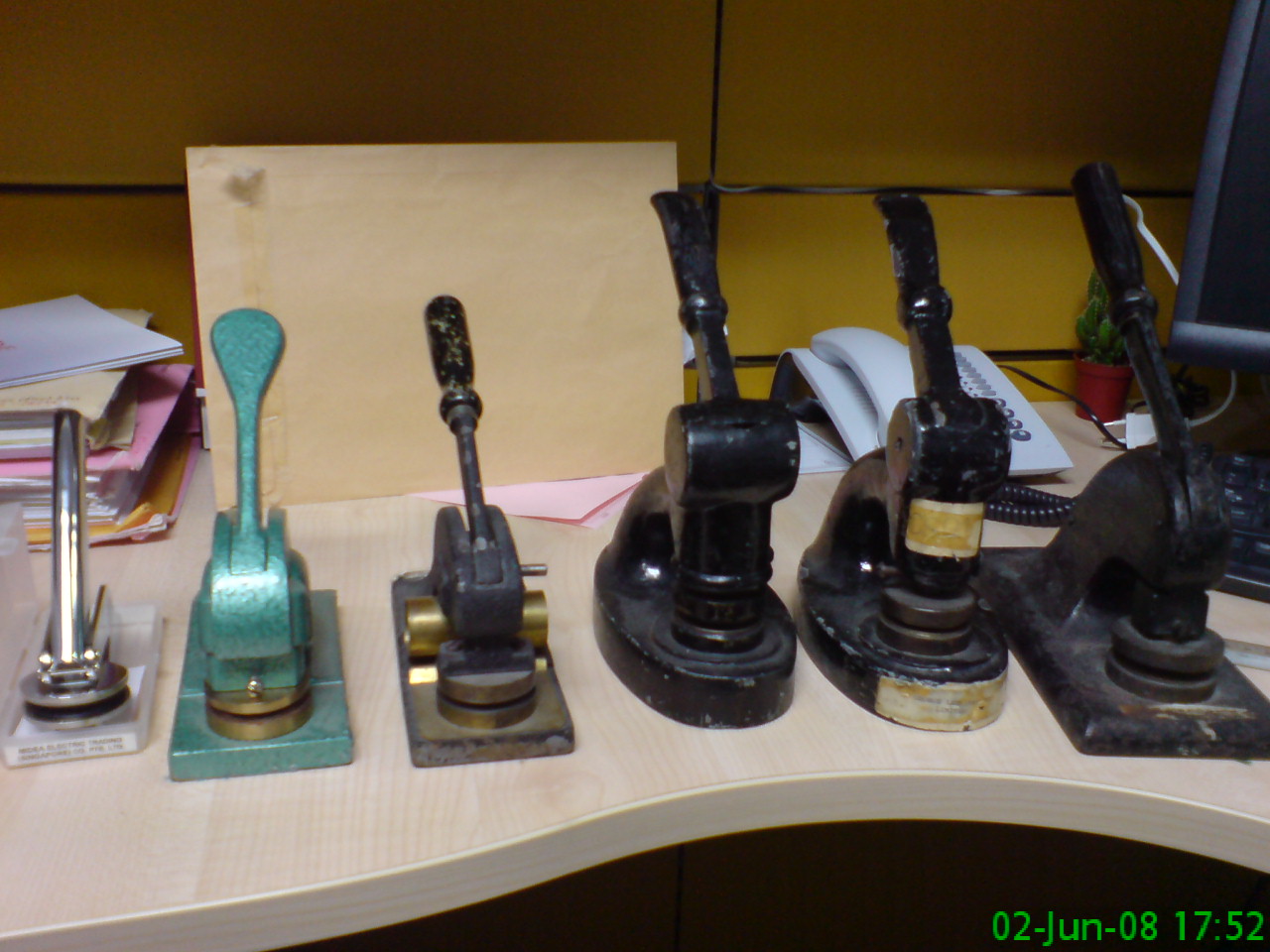This photo showcases a collection of six vintage seal embossing machines, traditionally used to create official raised seals on documents. The machines, aligned on a countertop, are arranged in a progression from right to left, illustrating the evolution of their design. On the far right, there is a large, clunky, and rusty machine made of wrought iron with a rectangular base, suggesting it is the oldest. Next to it is another aging machine with an oval base. As we move leftward, the machines become increasingly refined, culminating in a sleek, modern-looking embossing machine made of stainless steel on the far left. The machines are of various colors including black, black and brown, black and gold, blue and gold, and silver. Notably, one of the machines has a green body. 

Behind the machines, the background reveals an office setting with a cubicle wall, a multi-line office phone, and a small flower plant. Additional office supplies and documents rest on the countertop, including a light brown envelope with pink papers, a pink file, a brown folder, and a white folder. A desktop screen and keyboard are partially visible at the top right corner of the image. The photo is timestamped at the bottom right, indicating the date 02 June 08 and the time 1752, written in green.